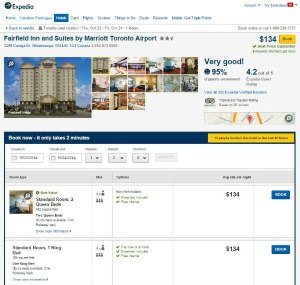This image is a screenshot from the Expedia website, showcasing rooms available at the Fairfield Inn and Suites by Marriott Toronto Airport. Despite some blurry text at the top, the primary information is clearly visible. Prominently displayed is the hotel's name along with its location in Toronto. A picture of the hotel reveals a mid-rise building with about six or seven stories. The ground floor features a lobby entrance with a distinctive green archway and glass doors, adjacent to a visible parking lot.

The user interface includes 15 clickable buttons for viewing various interior images of the hotel. On the right side, essential booking details are provided: the nightly rate is $134, with a yellow button available to proceed with the reservation. The hotel boasts a "Very Good" rating, scored at 4.2 out of 5, and a high satisfaction rate of 95%.

Further down, a menu offers a choice between two room types: a standard room with two queen beds and a standard room with one king bed. Each room's capacity and features are listed in a second column, and both options are priced at $134 per night. A blue button is available to finalize the booking for each room type.